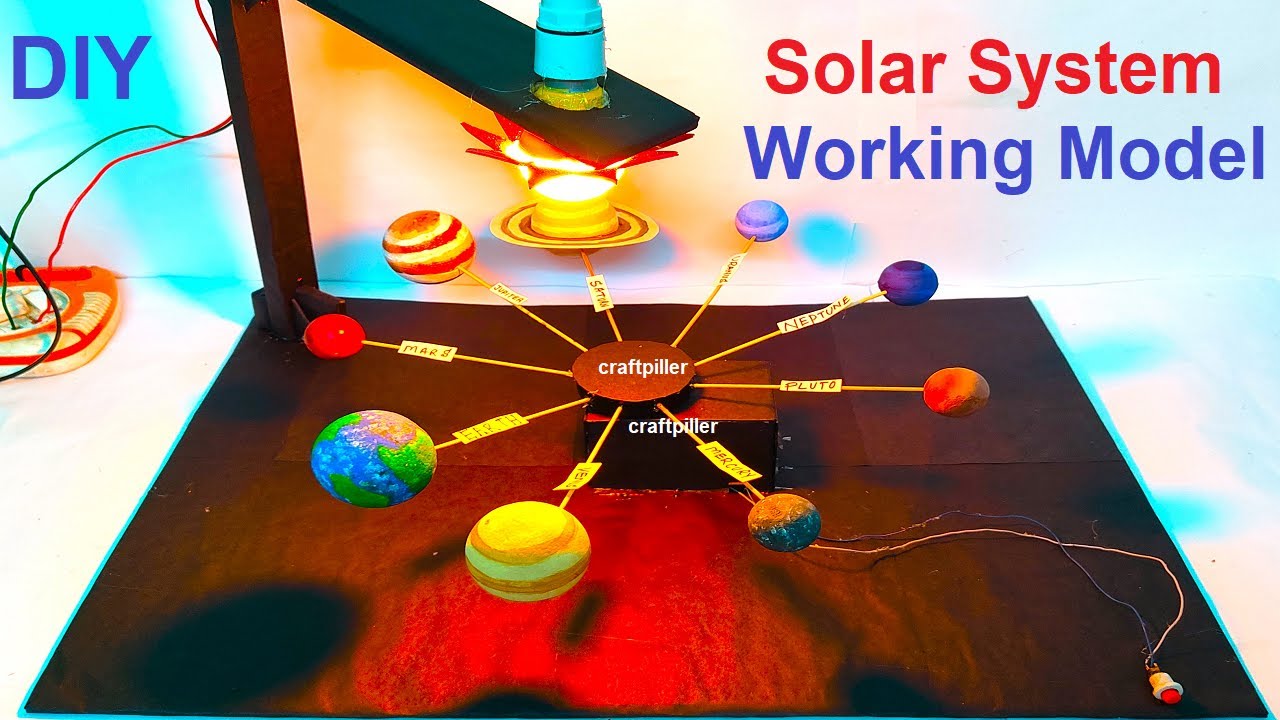This is a detailed 3D diagram of a DIY working model of the Solar System. In the top left corner, "DIY" is written in blue text, and in the top right corner, "Solar System" is written in red, followed by "Working Model" in blue. The model features labeled planets mounted on sticks that radiate from a central cardboard structure, labeled "Craft Pillar". Each stick represents a different planet, scaled to size with Earth being bright green and blue. Above the planets, a lamp with a sun motif is affixed to two wooden blocks, casting light downwards. From the base, two wires extend from a box with a red button, adding an electrical element to the model. The entire setup appears to mimic the planetary motion around the Sun, creating an educational and interactive depiction of the solar system.